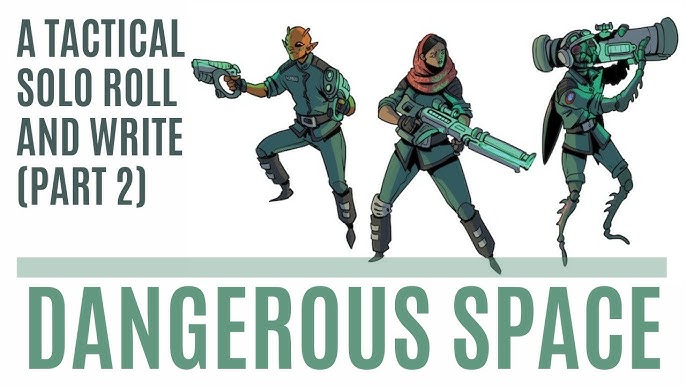This advertisement features a vividly animated, turquoise-blue color scheme and portrays three distinct, video game–styled characters equipped with various futuristic weapons. From right to left, the characters occupy three-fourths of the image. 

On the far right is an insect-like creature holding a sizeable rocket launcher. This character has reptilian features and limbs, blending seamlessly with its oversized weapon, making its face somewhat hidden.

In the middle stands a female character dressed in a green suit and wearing a Middle Eastern headscarf, or hijab. She wields the largest firearm among the trio, a powerful and futuristic long rifle, conveying an air of readiness and strength.

The character on the left appears to be an alien with elongated, pointed ears. Dressed in the same turquoise uniform, this alien holds two peculiar guns, suggesting a readiness for dual-wielding combat scenarios.

Set against this illustration, the text on the right of the image reads: "A Tactical Solo Role and Write [Part Two]." Beneath this, in the same color as the characters' uniforms, the title "Dangerous Space" is prominently displayed, completing the cohesive and dynamic advertisement. The overall aesthetic resembles a graphic novel or video game cover, encapsulating a sense of excited anticipation and impending action.